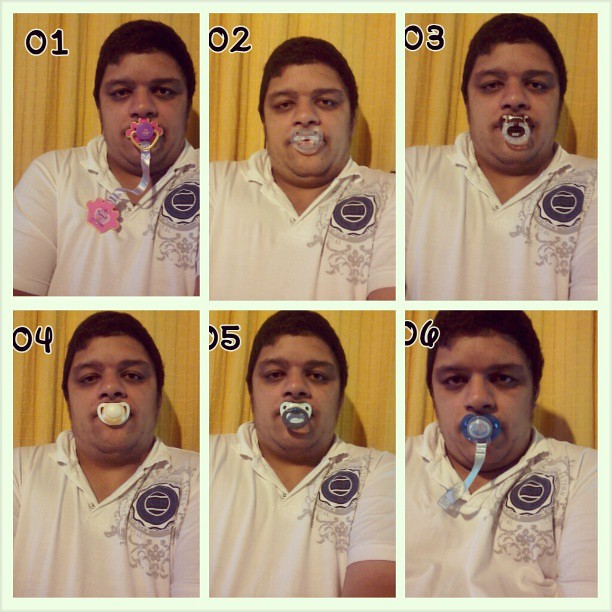This image is a vibrant, square-format color photograph arranged as a collage of six individual pictures, displayed in two rows and three columns. The photos showcase a middle-aged, dark-haired South Asian man with a clean-cut appearance, wearing a white open-neck collared shirt adorned with a small navy-blue emblem. He stands against a yellow backdrop, and each photo captures him looking seriously at the camera with a pacifier in his mouth. The pacifiers change slightly in each consecutive photo: the first picture (top left, labeled O1) shows him with a pink pacifier clipped to his shirt with a ribbon; the second photo (O2) features a clear pacifier, also clipped. The third image (O3) presents a golden pacifier with a ring. In the fourth photo (O4), he has a white pacifier, followed by a blue and navy pacifier in the fifth picture (O5). The final image (O6) displays a royal blue pacifier attached to a blue ribbon, clipped onto his shirt. The man's expression remains consistently serious across all six images, adding a humorous contrast to the whimsical presence of the pacifiers.